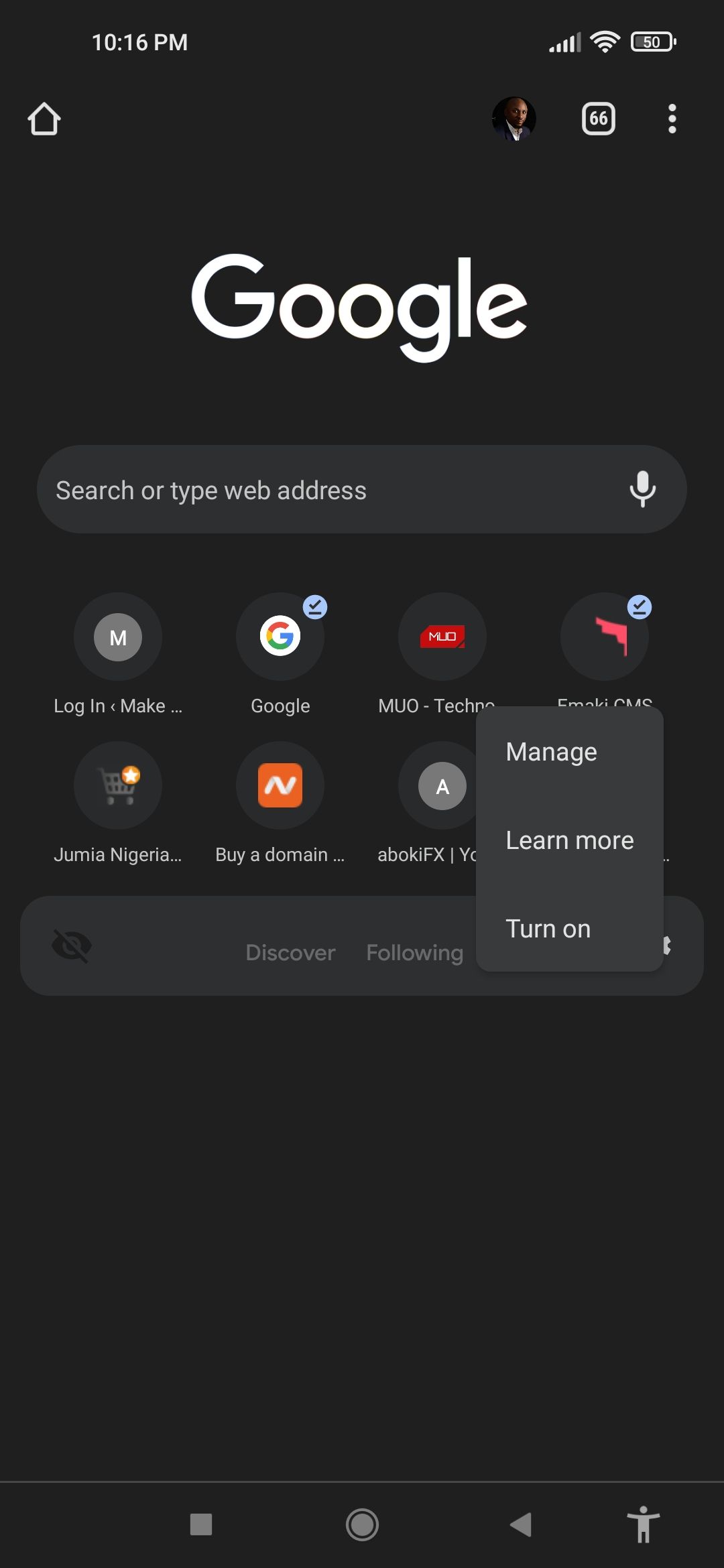Screenshot of the Google App on an Android Device in Dark Mode

This image captures a screenshot of the Google app on an Android device set to dark mode, taken at 10:16 p.m. according to the time displayed in the top left corner. On the top right, the status bar shows full Wi-Fi connectivity and a phone battery at 50 percent. The top left corner also features a profile picture of a man and a home button icon. Adjacent to these is an icon showing 66 open tabs and the vertical three-dot menu icon.

Below the status bar, the Google logo appears prominently in white. Beneath the logo is the search bar where users can input search queries or web addresses. Below this are a series of saved pin tabs labeled "login," "Google," "MUO," an obscured tab, "Biodomain," and a highlighted tab. Options reading "manage," "learn more," and "turn on" are positioned nearby.

At the very bottom of the screen reside the navigation buttons and a partially visible bar indicating the Discover and Following features, which are currently turned off.